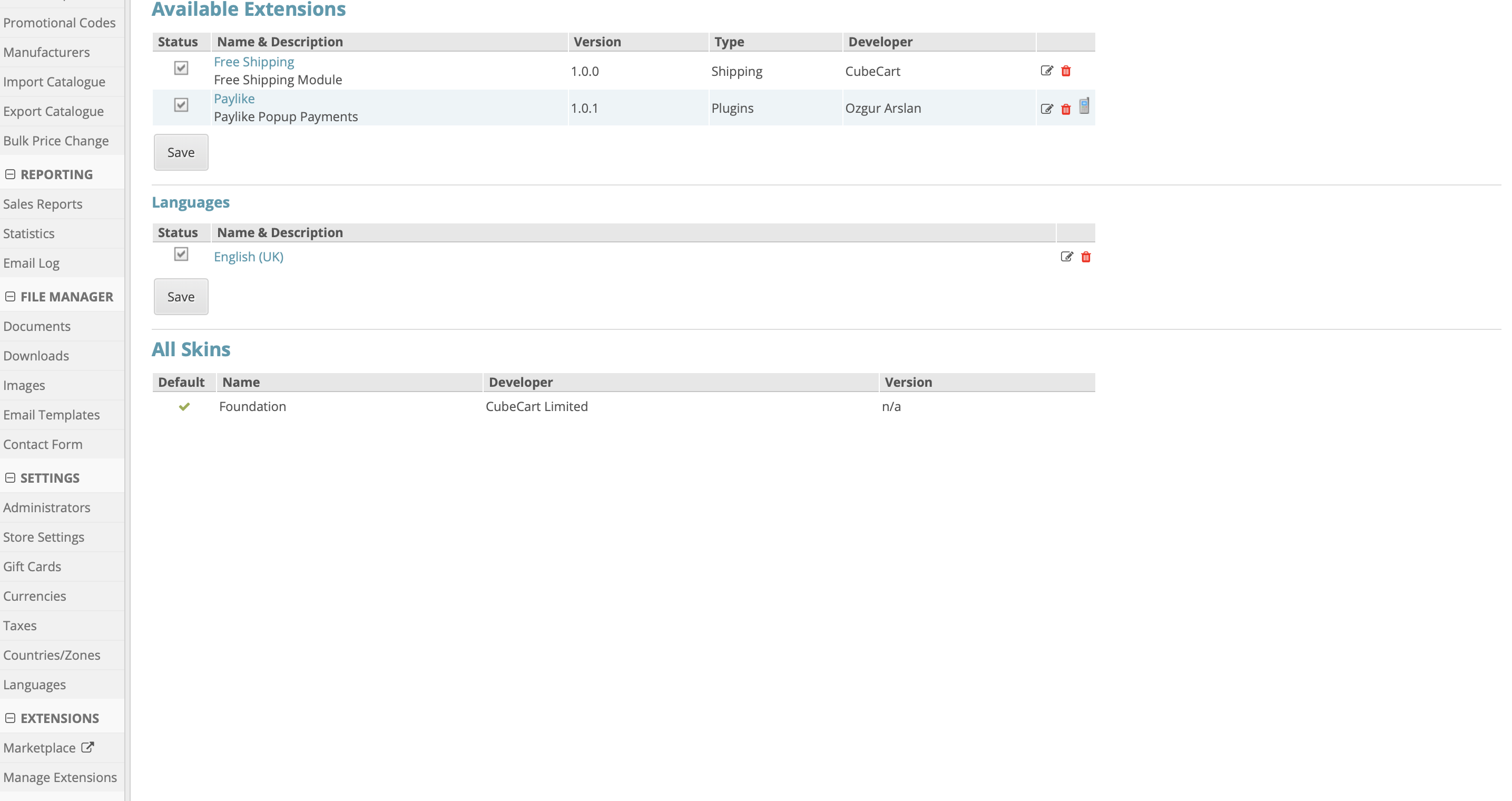This image is a detailed screenshot of a website building interface, specifically showcasing the available extensions tab. At the top of the page, the tab is titled "Available Extensions" in prominent blue, bold text. The layout features a vertical gray sidebar panel on the left, which contains a list of expandable categories. The categories listed are: "Promotional Codes and Manufacturers," "Import Catalog," "Export Catalog," "Bulk Price Change," and a category named "Reporting" that includes options to minimize or maximize the section. Within the "Reporting" category, there are sub-items: "Sales Reports," "Statistics," and "Email Log." Further down, additional categories such as "File Manager," "Settings," and "Extensions" are listed.

On the right side of the interface, below the "Available Extensions" header, a horizontal gray banner displays multiple column headers: "Status" on the left, followed by "Name and Description," "Version," "Type," "Developer," and a partially visible section featuring a checkbox icon and a red trash can icon on the far right. Underneath the "Name and Description" section, there is a "Save" button to the left. The interface also mentions "Languages" and "All Skins," though their exact placement is unspecified in the description.